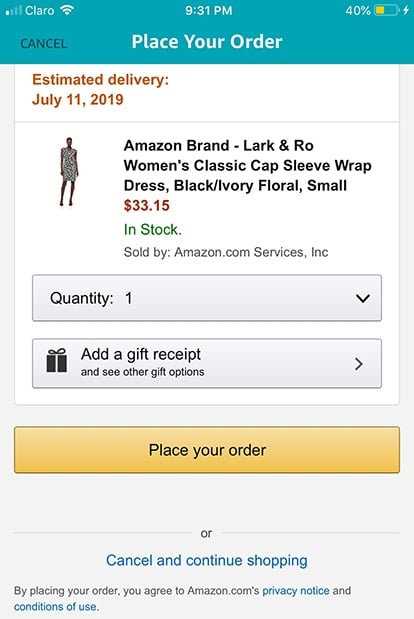The image captures a screenshot of an Amazon checkout page on a smartphone. At the top of the screen, there is a teal-colored status bar displaying various icons: the Claro network signal bars, WiFi signal bars, "3Q" with an unreadable part, the time "9:31 PM", and a battery icon at 40%. Below the status bar, a yellow section features "Cancel" on the left, and "Place Your Order" in the center.

The main body of the screenshot details the order information. The delivery estimate reads "Estimated delivery: July 11, 2019." Directly below, the product description states, "Amazon Brand - Lark & Ro Women's Classic Cap Sleeve Wrap Dress, Ivory/Black Floral, Small, $33.15. In Stock, Sold by Amazon.com Services, Inc." This section also shows the quantity set to one, with additional options accessible via a dropdown menu labeled "Add gift receipt / See other gift options."

The "Place Your Order" button is prominently displayed in an orange bar with black text, spanning the width of the screen. Underneath this bar, there's a horizontal line separating it from a "Cancel and Continue Shopping" link in blue, alongside a note about agreeing to Amazon's Privacy Notice and Conditions of Use upon placing the order.